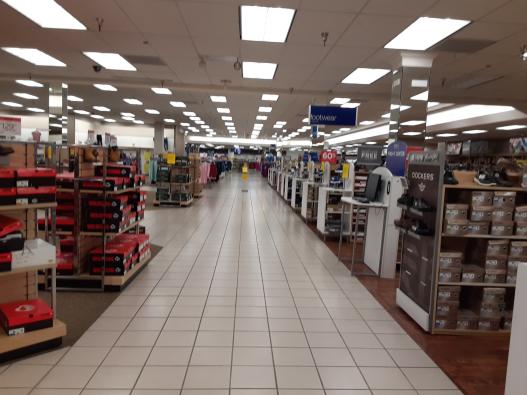This photograph captures a main aisle of a clothing and shoe store, reminiscent of a Kohl's. The right side features a display of shoes prominently marked by a "Dockers" sign, suggesting this is indeed a shoe section. Shoe boxes are also visible on the left side of the aisle. The floor consists of white and beige-colored tiles, and the ceiling is adorned with built-in long fluorescent lights that illuminate the scene. A large blue sign hangs above, though the wording on it is not legible. The clean and organized layout directs the viewer's gaze straight down the aisle, providing a clear view of the store's interior.